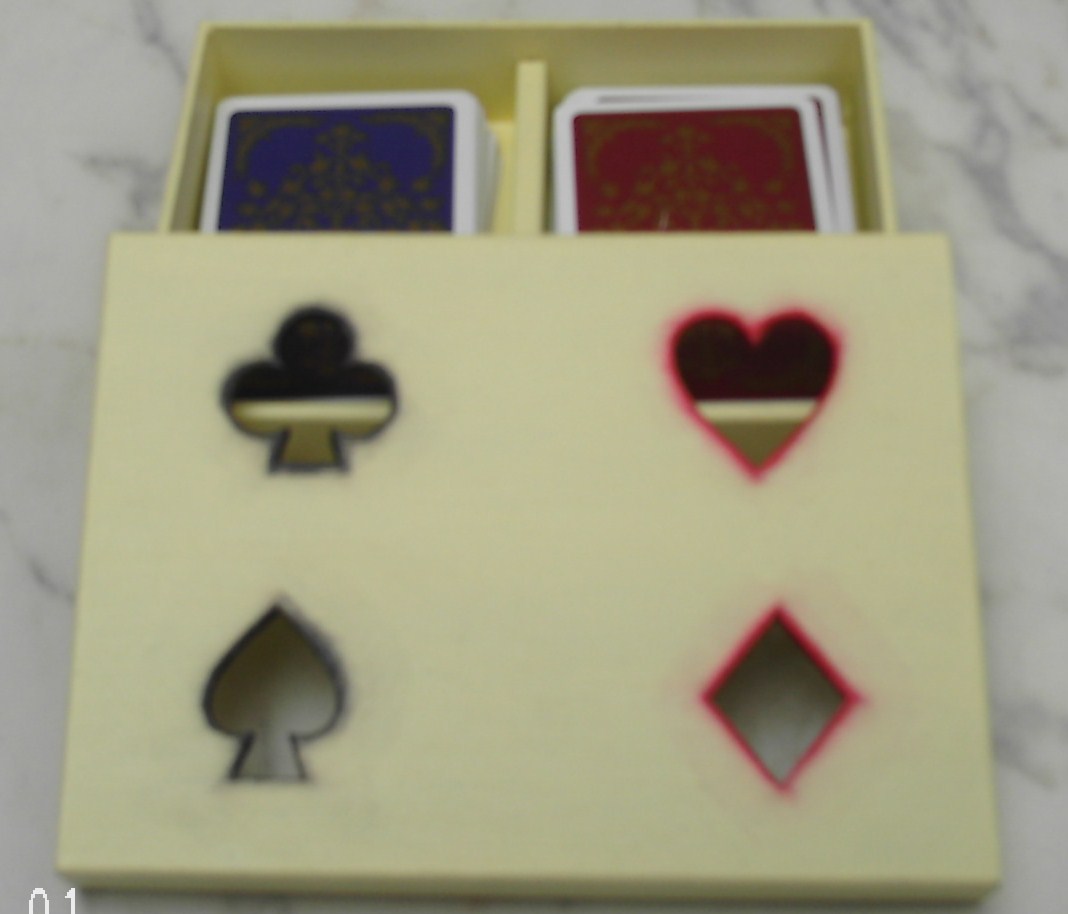On a white and gray marbled countertop sits an elegant wooden container designed to hold two decks of cards. The container, crafted from light beige wood, features a small drawer that smoothly pulls out, revealing a neatly divided interior. The top of the container is decorated with intricately designed club and spade symbols, each outlined in black, positioned at the top and bottom. On the opposite side, heart and diamond symbols, outlined in red, are similarly arranged. 

Inside the drawer, which has a light yellow tint, are two distinct decks of cards. One deck is predominantly blue and black, while the other deck is red and gold. Both decks are bordered in white, adding a touch of elegance. The red and gold deck is adorned with delicate gold-leaf patterns, while the blue and black deck features gold and black leaf designs against the rich blue background. This charming container not only organizes the cards but also adds a stylish touch to any setting.